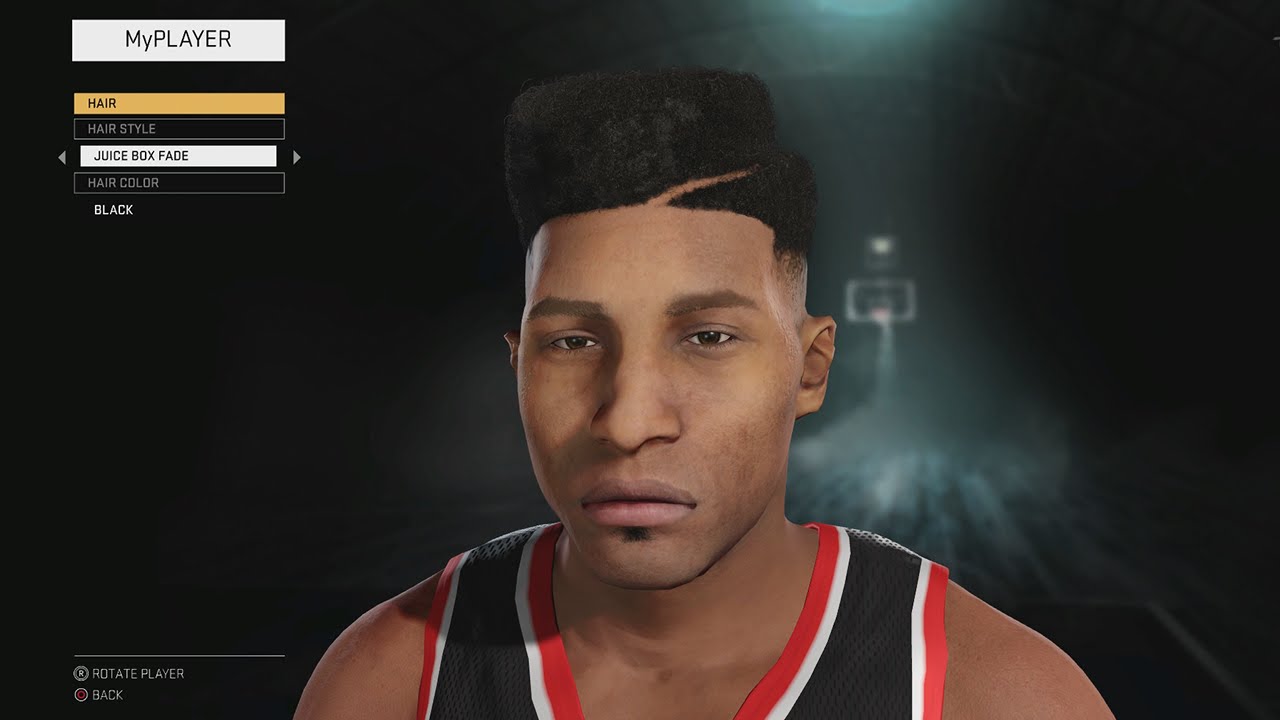A screenshot from a video game character creation interface, generated by AI, is displayed. The interface prominently features headings in various colored boxes. At the top, a yellow box is labeled "Hair," a black box reads "Hair Style," and a white box is marked "Hair Color." The selected hair color is black, as indicated below in another black box. Instructions for rotating the character and navigating back are shown on the screen, suggesting user interactivity.

The character being customized is a male figure with hair closely shaven down to the scalp, save for a styled swish on the top. Notably, his ears have a distinctive, unusual shape. Clothing details include an orange trim around the neck, a white stripe, and a brown V-neck shirt. In the distant background, the faint outline of a light and a basketball hoop can be seen, hinting at a sports-themed setting.